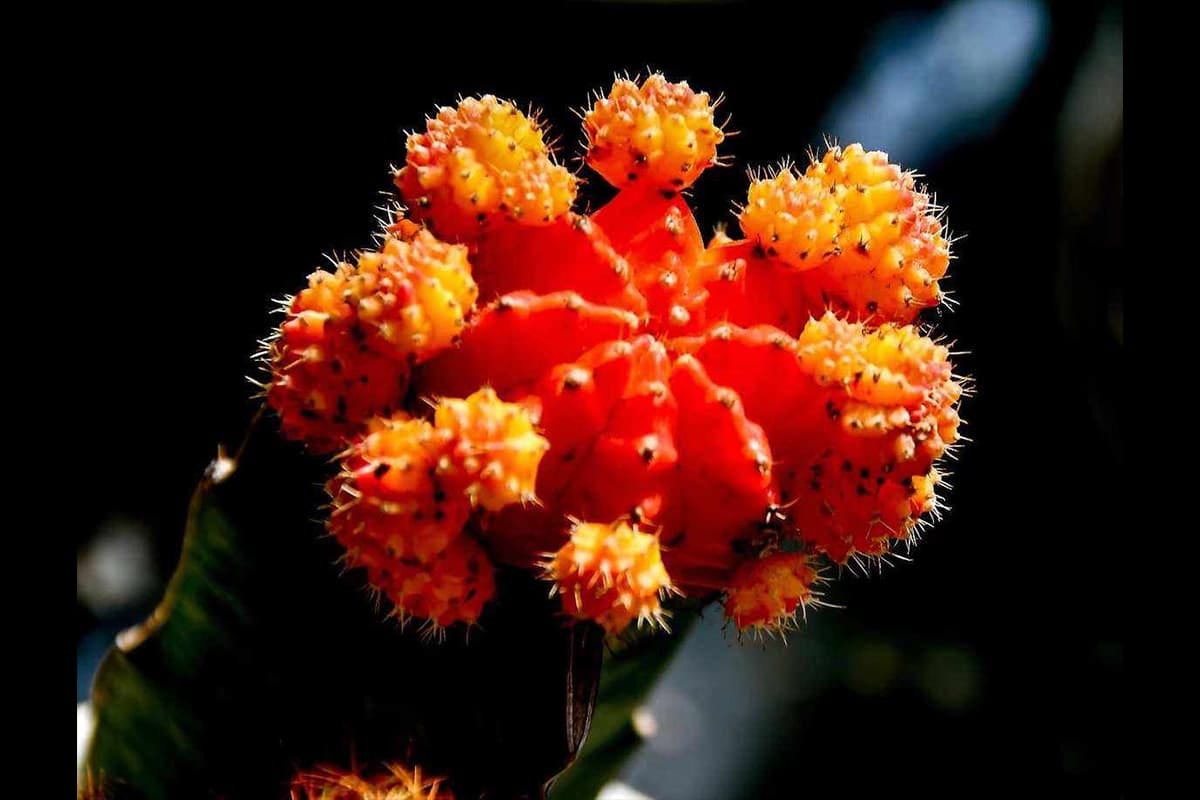In the image, set against a dark, blurred blackish background with a faint streak of light in the top right corner, is a close-up of a vibrant cactus. The cactus extends diagonally from the bottom left, distinguished by its deep green color and tiny stickers. Dominating the frame is the cactus flower, vividly lit as if under a spotlight. This striking flower forms a brilliant sunburst pattern at the top, featuring a deep, vivid orange center that divides into eight sections. Surrounding this central bloom are smaller growths in hues of yellow and gold, each densely covered in tiny white spines resembling little hairs. These offshoots create a spiky, almost pin cushion-like appearance, adding to the intricate texture of the scene. The flower and its growths give a vivid, spiky visual experience that seems to leap from the darkness.